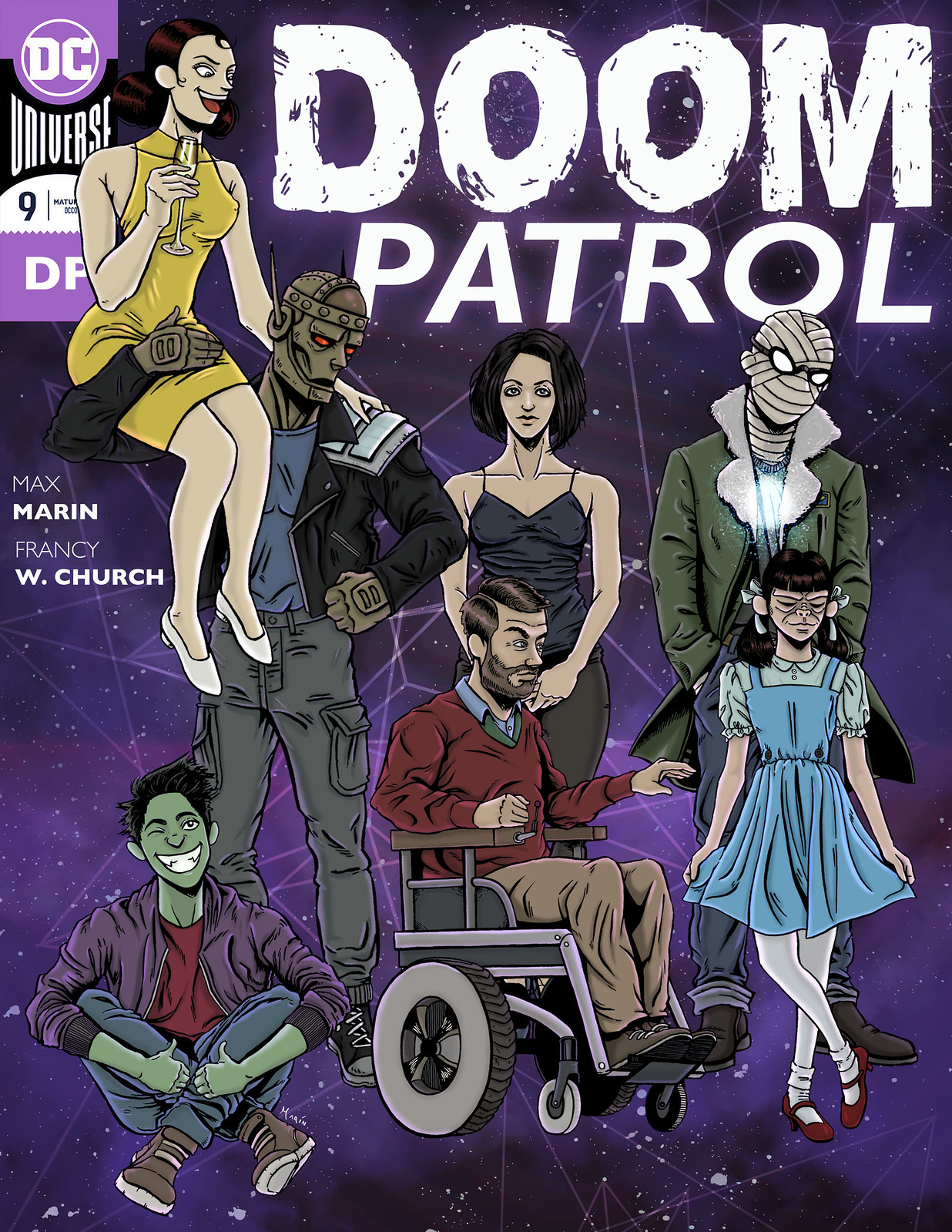The front cover of a comic book, titled "Doom Patrol" in etched white letters in the top right, presents a vivid space-like background in blue and purple, adorned with small white stars and interconnected by light purple geometric lines. In the top left corner, "DC Universe Nine" is displayed in purple and white within a small card-like column. Below that, the names Max Morin and Francie W. Church appear, with surnames in bold white.

The centerpiece showcases seven diverse characters: 

1. At the bottom left, a youthful character with green skin, green hair, and a purple jacket, smiling as he sits cross-legged.
2. Positioned centrally, a male figure in a red sweater, sitting in a wheelchair, extending one arm outward.
3. To the middle left, a woman in a yellow dress is riding on the shoulders of a man wearing a leather jacket, whose head is encased in a metal helmet.
4. Directly right of the metal-headed man stands a woman with black hair, dressed in a black outfit.
5. Behind this group, towards the right, a figure in a long green coat with bandages covering his face and goggles, exuding a mummy-like appearance.
6. Nearby, to the right, a monkey-like character donned in a blue dress, smiling with eyes closed.

The meticulously illustrated cover page not only captivates with its vibrant and dynamic ensemble cast but also with its intriguing interstellar backdrop, setting an adventurous tone for the comic within.